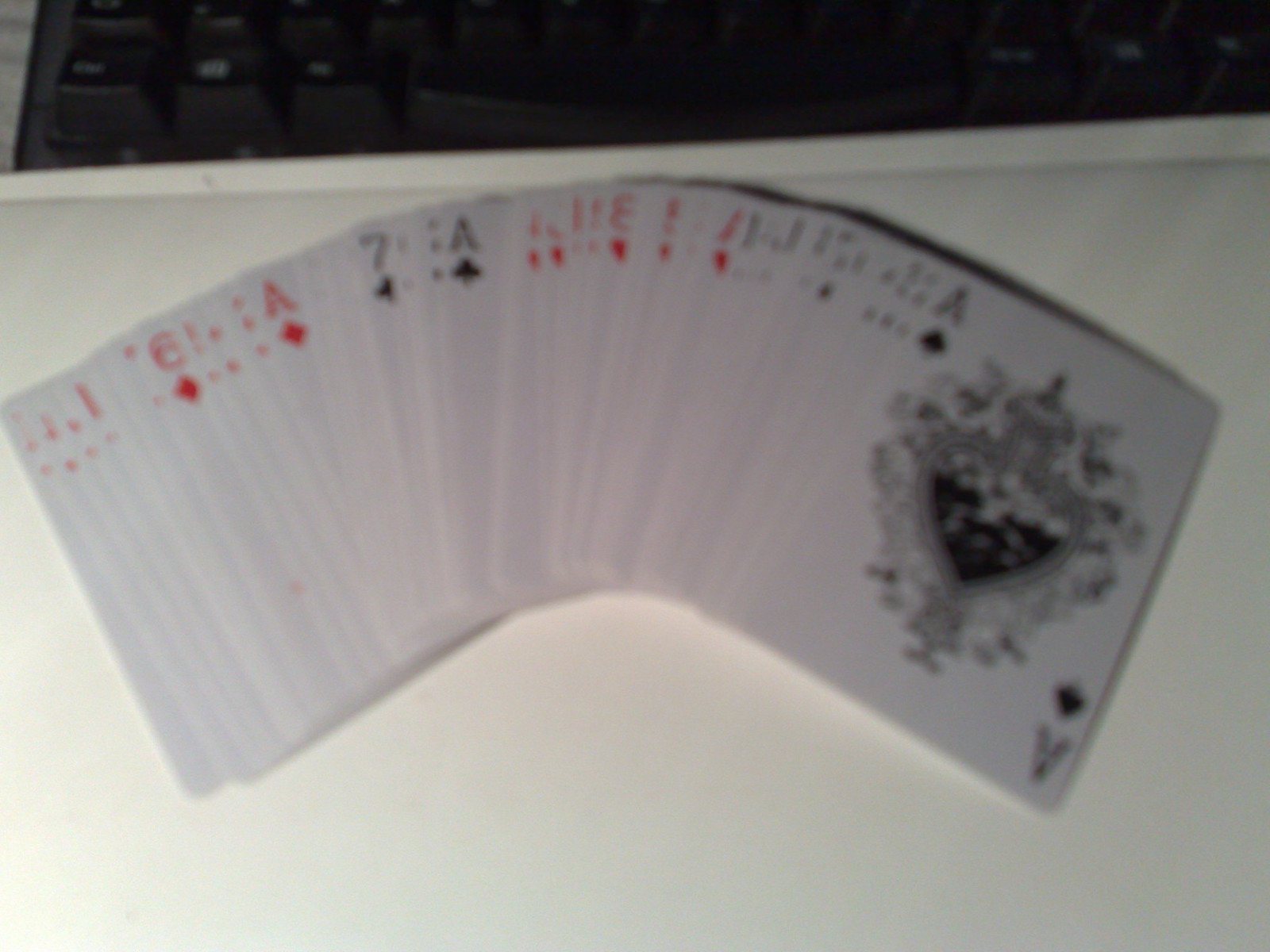A fanned deck of cards is arranged on a white countertop, illuminated subtly at the bottom left in an otherwise dark room. The cards, mostly out of focus, reveal glimpses of individual entries: the six of diamonds, the ace of diamonds, the seven of clubs, and the eight of clubs are slightly visible, along with the eight and ace of hearts. At the far right, the ace of spades stands out with its intricate design. The card's face features a large black spade symbol, the bottom 80% shaded in black and the top in white. The design extends upwards like a bottle with a pointed cap, surrounded by an ornate floral pattern of vines. The text "Ace of Spades" appears at the bottom right of the card.